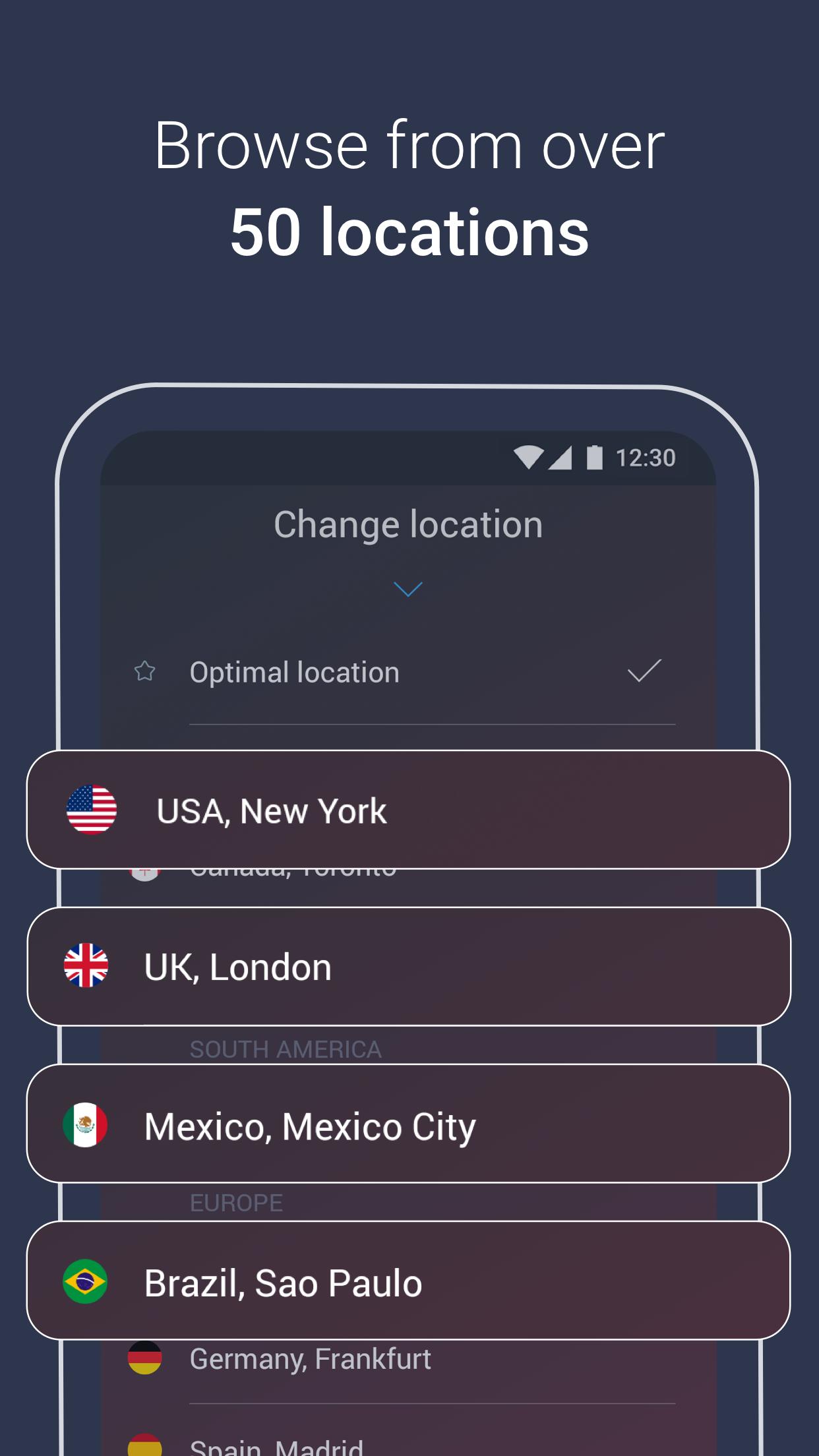A screenshot from a smartphone displaying a VPN app interface. The app background is dark blue, and the layout is vertically oriented. At the top, in white text with varying thickness, it says, "Browse from over 50 locations," with "50 locations" in a bolder font. Below, an illustrated outline of a phone shows standard icons like Wi-Fi, signal bars, battery status, and the time, 12:30. The banner at the top within the app reads "Change Location" with a small blue arrow, followed by "Optimal Location" marked with a check mark and a star. Below, four prominent location options are visible: 

1. "USA, New York" with an American flag.
2. "UK, London" with a British flag.
3. "Mexico, Mexico City" with a Mexican flag.
4. "Brazil, Sao Paulo" with a Brazilian flag.

In the background, smaller text lists additional locations: "Germany, Frankfurt" and "Spain, Madrid."